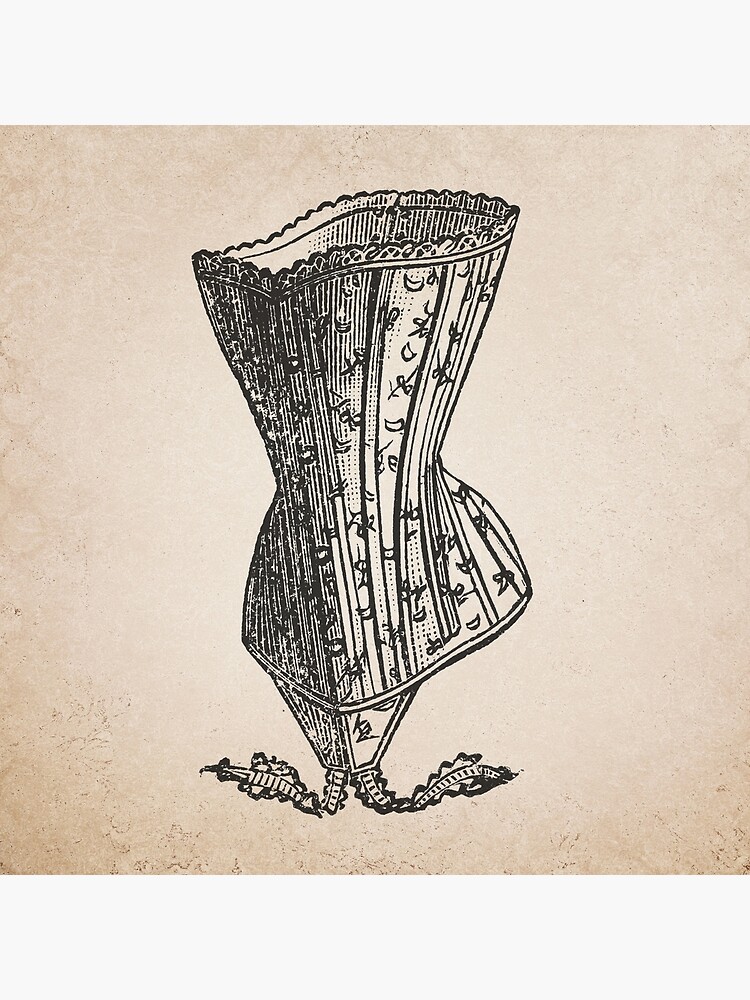The illustration appears to be a detailed diagram of a corset, drawn in black ink on aged parchment paper, creating a light beige to dark brown background that appears crusty, as if stained or dirtied over time. The corset itself is a form-fitting garment designed to shape the body, depicted with a prominent color scheme: black on the left side and white on the right. It features intricate, vertical line decorations possibly representing leaves, moons, and flowers. The garment elegantly curves to fit the bust, waist, and hips, with two small flaps and ties descending from the front. The waist and top areas are clearly defined, and there are slats running vertically, suggesting the supportive structure. The bottom of the corset includes straps that would wrap around the legs, designed to hold the corset securely in place when worn.